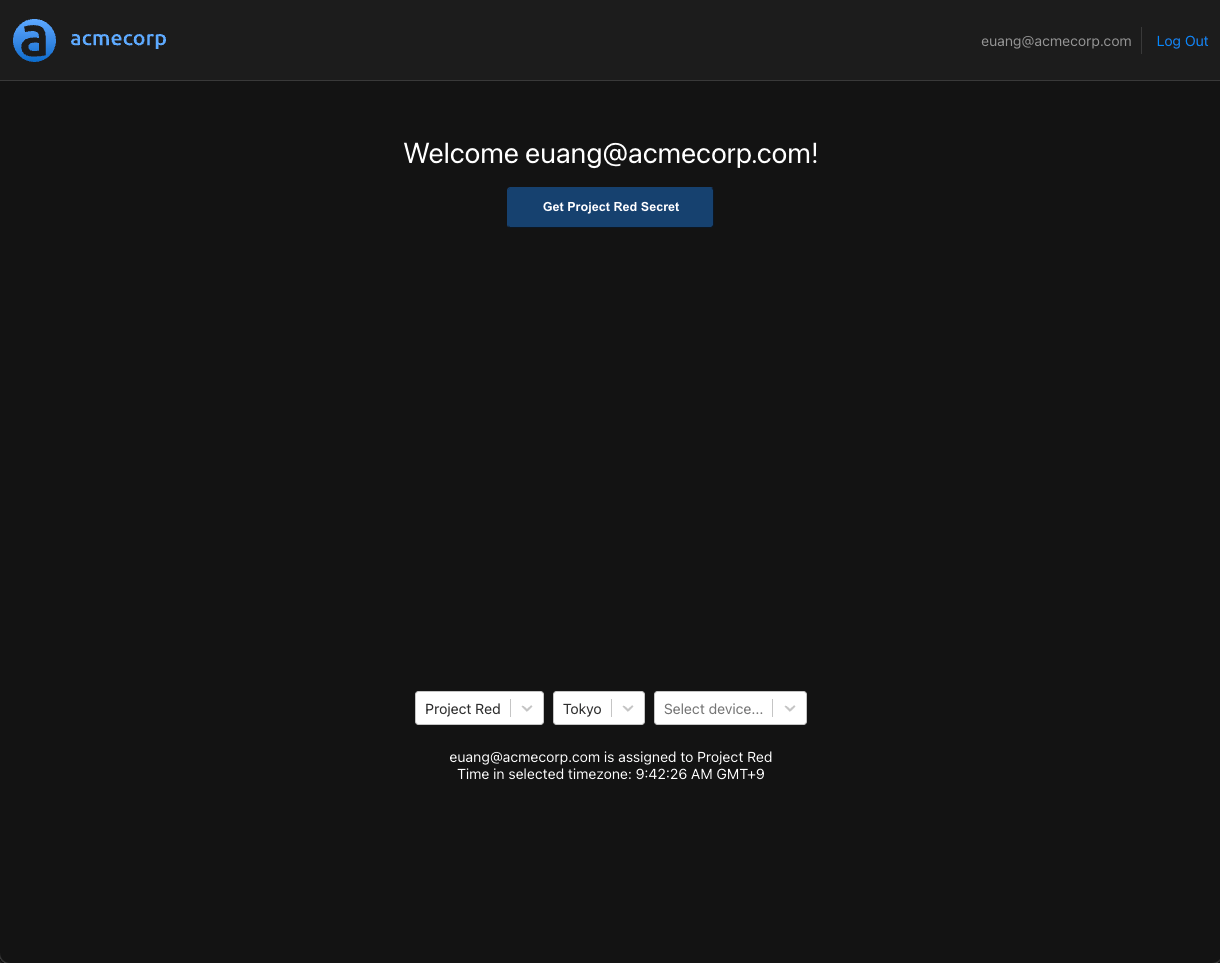This image captures a website interface set against a black background. In the top left corner, a lowercase 'a' enclosed in a blue circle marks the logo, with the company name "ACMECORP" written adjacent in matching blue font. To the right, an email address, "EUANG@ACMECORP.com," is displayed, alongside a logout link. Directly below, in prominent white font, the text "Welcome, EUANG@ACMECORP.com!" cheerfully greets the user. Beneath the greeting, a conspicuous blue button labeled "Get Project Red Secret" stands out. Continuing downward, the phrase "Project Red" is written. On the right side of the interface, the text indicates "Tokyo" as the selected location and prompts the user to choose a device. The current time in the selected time zone is displayed as "9:42:26 AM GMT-9."